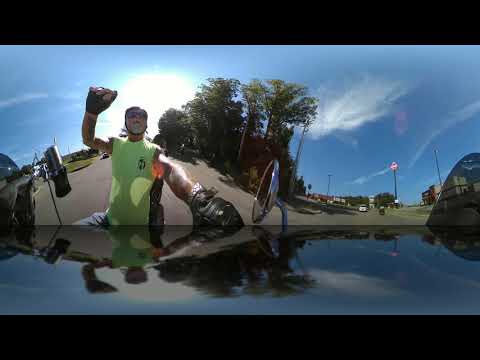In this detailed image, we see a man wearing a yellow tank top and sunglasses, equipped with hand gloves and a helmet, ensuring his safety as he engages with a vehicle. His left wrist sports a watch, and his left hand firmly grips the side mirror of the vehicle, while his right hand is raised in a fist, as though reacting to something or celebrating. The scene is set outdoors on a sunny day, evidenced by the bright light and scattered clouds in the sky. The backdrop consists of trees and distant buildings, contributing to a landscape that slopes downward into what looks like the bottom of a hill. The image is taken from an unusual perspective, possibly from a camera attached to the back of the vehicle, giving a wide-angle view that distorts some elements. Despite the graininess of the photo, the context provides a vivid depiction of the man amidst this lively and somewhat dynamic setting on the road.